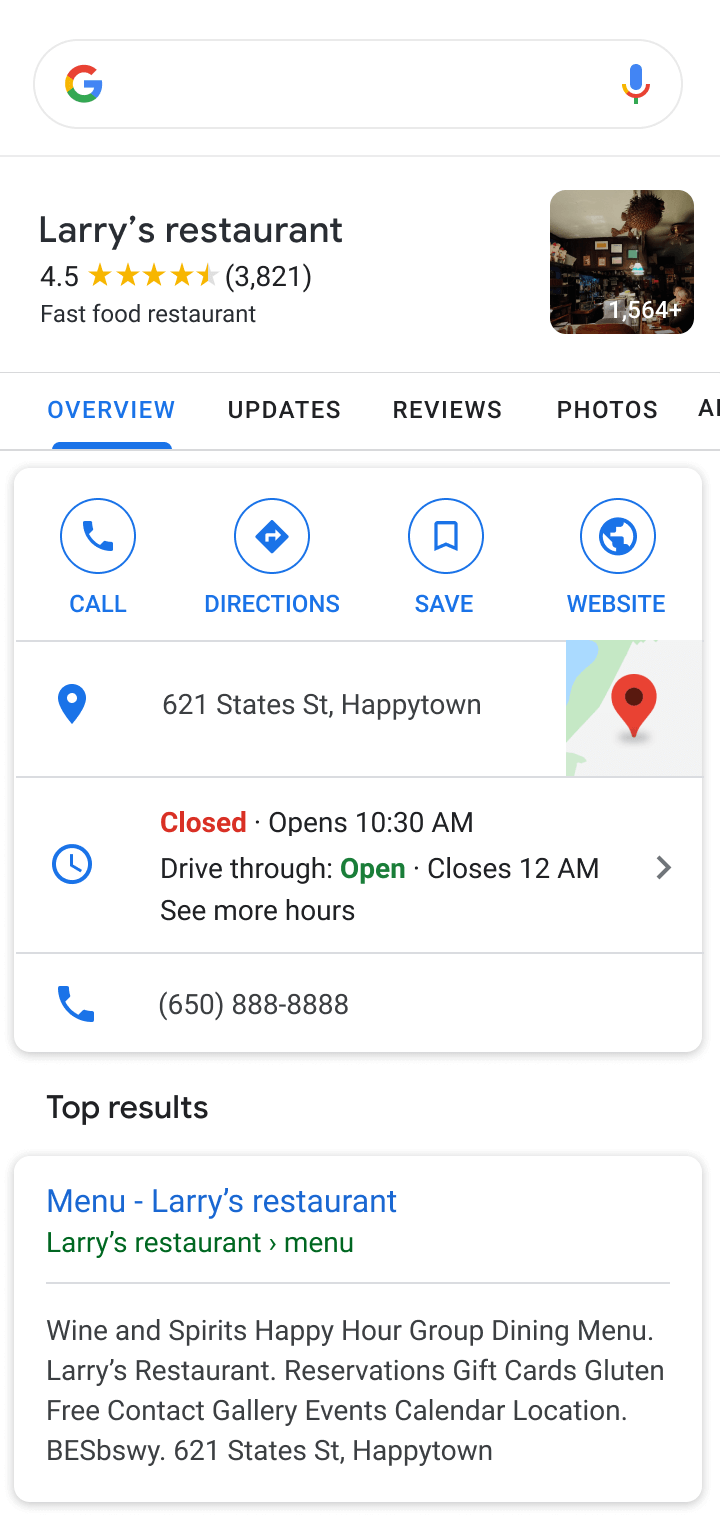In this image, we see a Google search results page prominently featuring Larry's Restaurant. At the very top, the recognizable Google logo is visible to the left of the search bar, which has a voice input button situated on its right side. Below the search bar, a comprehensive listing for Larry's Restaurant appears, highlighting its 4.5-star rating based on 3,821 reviews. Identified as a fast food restaurant, the following categories and information are detailed: Overview, Updates, Reviews, and Photos. Navigation options labeled "Directions" are present as well.

The restaurant's address is listed as 621 States, Happy Town. It is currently closed but will open at 10:30 AM. The information also includes references to additional offerings such as wine and spirits, happy hour specials, and a group dining menu. Other features mentioned are the ability to make reservations, purchase gift cards, and options for gluten-free dining. Additionally, tabs for Contact, Gallery, Events, Calendar, and Location provide further details about the restaurant.